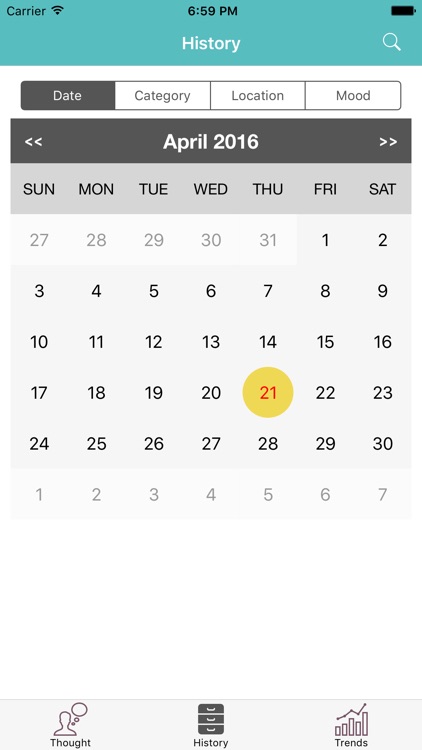Screenshot of a mobile calendar interface with a sleek design. The top section of the screen displays a full Wi-Fi signal, the time as 6:59 p.m., and a fully charged battery. The page is titled "History" against a green background, accompanied by a search bar. Below the title, there is a tab menu offering options to sort by Date, Category, Location, and Mood; the Date option is selected. 

The header of the calendar is dark gray and reads "April 2016." Beneath this, a lighter gray bar displays the days of the week. The calendar itself features a white background with black text, with dates from the previous month grayed out. The 21st of April, highlighted in red against a yellow background, falls on a Thursday and stands out prominently. April 1st starts on a Friday.